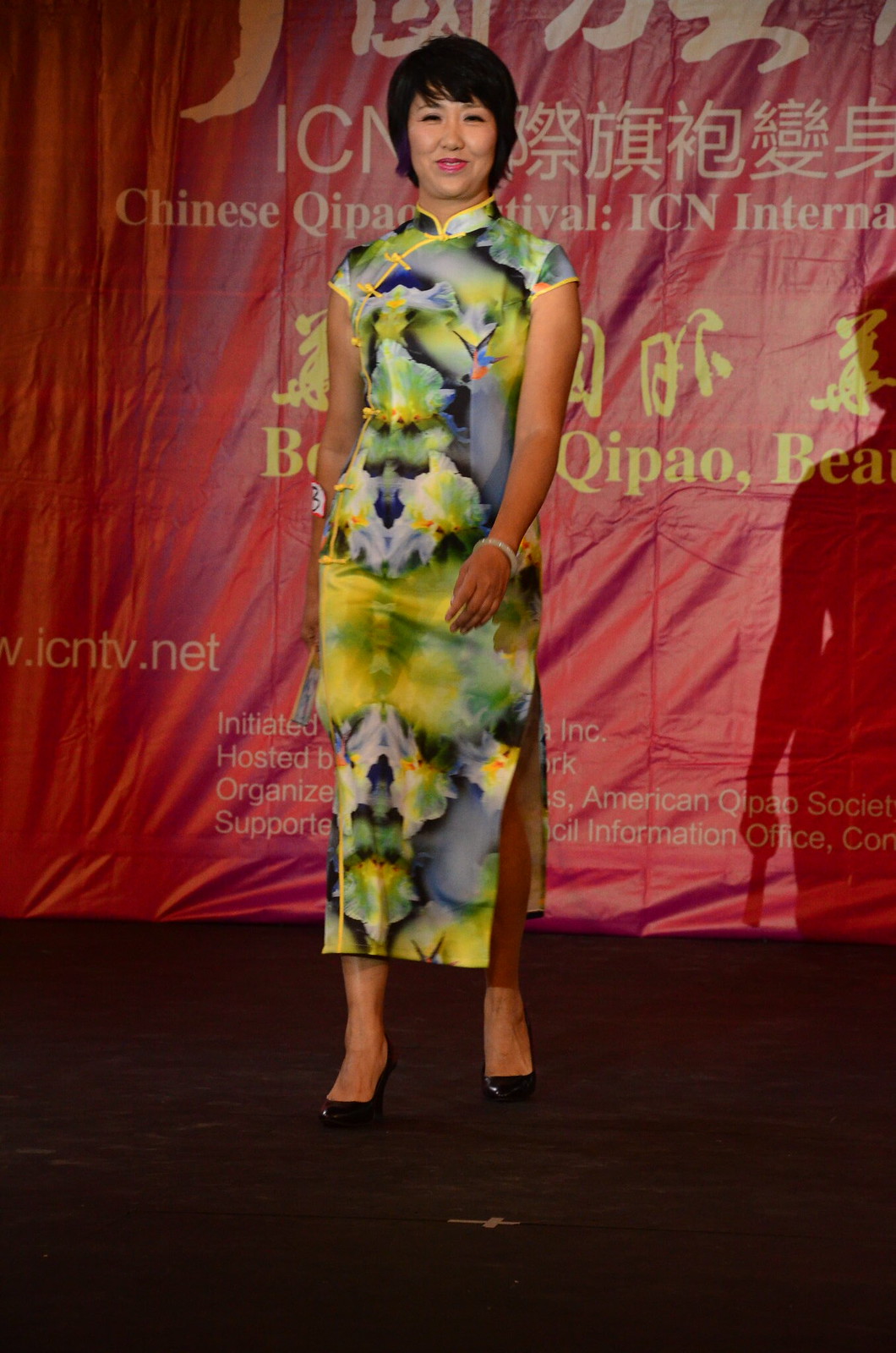The image features an Asian woman, possibly a celebrity or actress, smiling as she walks towards the camera on a black runway. She is standing against a large, reddish backdrop, which is adorned with Chinese text and partially visible English translations, including references to a Chinese Festival and the website www.icntv.net. The woman is dressed in a long, traditional Asian-style dress that is predominantly turquoise with a colorful pattern incorporating yellow, dark blue, and tie-dye elements. The dress reaches down to her ankles, and she is wearing black heels. Her hairstyle is short and black, approximately the length of her face. The red backdrop behind her has an ornate design, contributing to the grand and festive atmosphere of the scene.